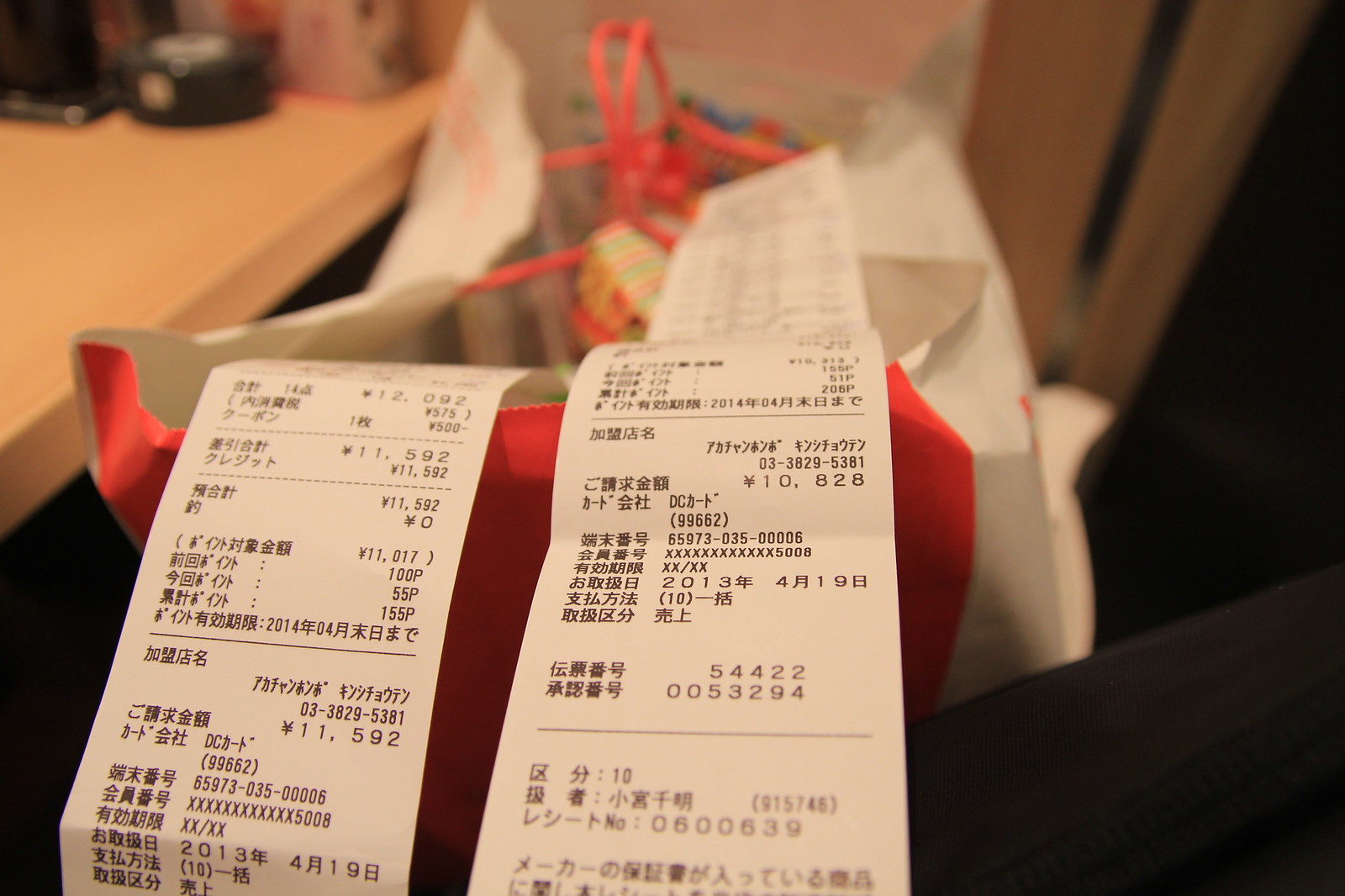The photograph depicts two long white receipts, predominantly featuring Japanese characters, positioned vertically and prominently in focus in the foreground. Both receipts are dated 2013 and contain numerous numerical details. These receipts are partially nestled over a red and white paper shopping bag with red handles, likely suggesting a recent purchase. The bag appears to contain some brightly colored, possibly striped, wrapped gifts. The background of the image is blurred, revealing hints of a home setting with a tan-colored table and wall, a black chair, and some indistinct black and pink objects on a countertop. Overall, the scene suggests a mixture of recent shopping and a cozy domestic environment.